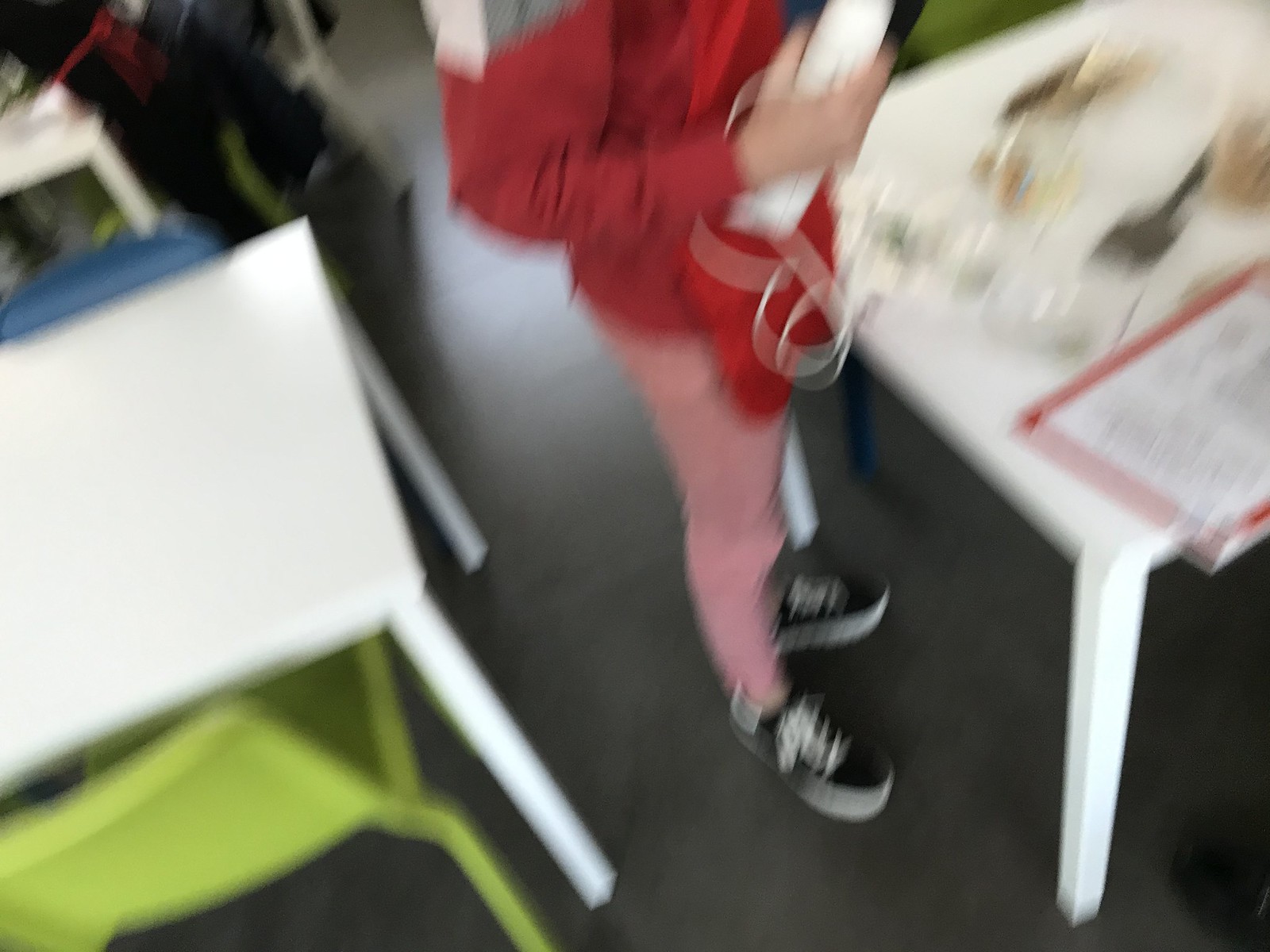In this blurred photograph, the viewer's focus is directed towards a classroom setting featuring an assortment of white desks and colorful chairs, including one blue and one vivid chartreuse green chair. Dominating the image's center is an individual adorned in black sneakers with white soles and laces, pink pants, and a red and white top. This person appears to be holding a long white object with an attached wire. 

To the right, a desk harbors a peculiar assortment of items, including something with a red outline and a white interior, possibly a bag, although the blurriness makes it difficult to ascertain. Additionally, the desk holds two black objects and a couple of indistinct brown items, their true forms obscured by the lack of clarity in the photograph. 

In the background, there is another individual clad in a dark gray coat over a black shirt, positioned near yet another white desk. The dark gray, seemingly concrete floor completes the scene, adding to the overall ambiance of the classroom.